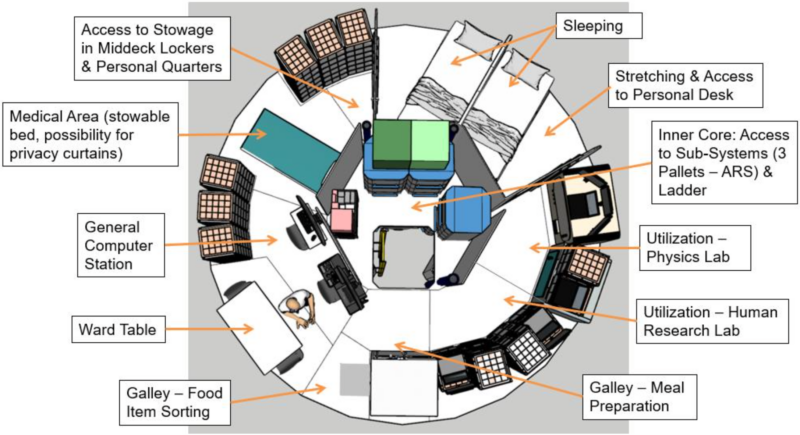This image is a detailed, circular blueprint of what appears to be a highly organized and multi-functional space, possibly resembling a spacecraft or specialized habitat. The background is gray, annotated with multiple labels and orange arrows pointing to various key areas within a white circle. Key sections include a galley for meal preparation and food item sorting, a ward table, a general computer station, and a medical area. There's a stowable bed highlighting the sleeping area, along with the possibility for privacy curtains nearby. Access is provided to stowage in mid-deck lockers and personal quarters. Other notable areas include points for stretching and access to a personal desk, an inner core for subsystem access, three pallets ARS, and a ladder. The image also marks specialized labs for utilization physics and human research. The meticulous design shows everything placed strategically, allowing individuals to smoothly transition from one function to another within the circular layout.